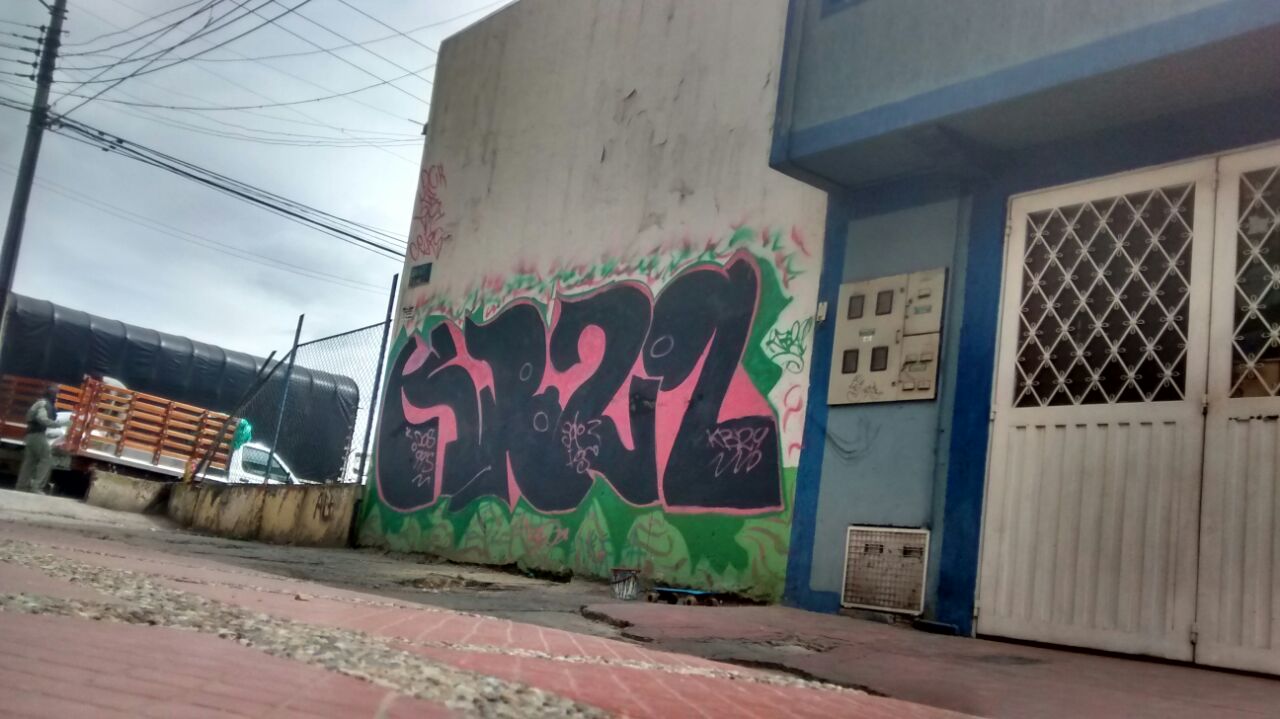This color photograph, taken in landscape orientation, features an older building in a commercial setting, viewed from the street. The exterior wall of the building is primarily a weathered white stucco with blue trim, including a blue canopy extending over the doorway from the bottom right corner. Underneath the canopy, two white wooden doors with diamond-shaped grids in metal frames provide entry. The wall is adorned with graffiti in black and pink, outlined in green, with green graffiti grass painted at the bottom. The graffiti features a mix of letters and numbers that are mostly illegible. 

In front of the building, the foreground showcases a red brick walkway interspersed with some stone and gravel, leading to a cement pad by the entrance. The scene includes a white truck parked to the left side of the image, with a man standing beside it. The truck has a wooden gate on its bed. Signs are posted on the left side of the building, and a telephone pole with wires extends toward the structure, indicating the presence of utility services. The overcast sky suggests a foggy or cloudy day, adding a muted tone to the scene.